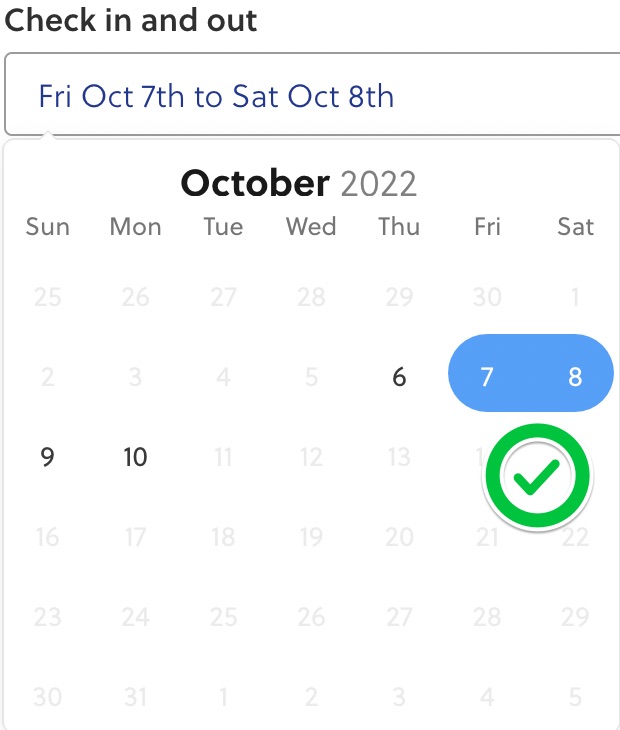The image showcases a calendar for the month of October 2022. At the top left-hand corner is a bold, black "Check-in/Check-out" label, with the "C" in "Check" capitalized. Directly below this label is a highlighted white bar with gray edging, containing text in a purple-blue font that reads "Fri-Oct-7th to Sat-Oct-8th," although part of the text is cut off on the right side. 

Below this bar lies the main calendar grid, displaying days of the week in the order of Sunday, Monday, Tuesday, Wednesday, Thursday, Friday, and Saturday. Notably, the dates "7th" and "8th" of October, corresponding to a Friday and Saturday, are encircled in blue, indicating a specific period of interest.